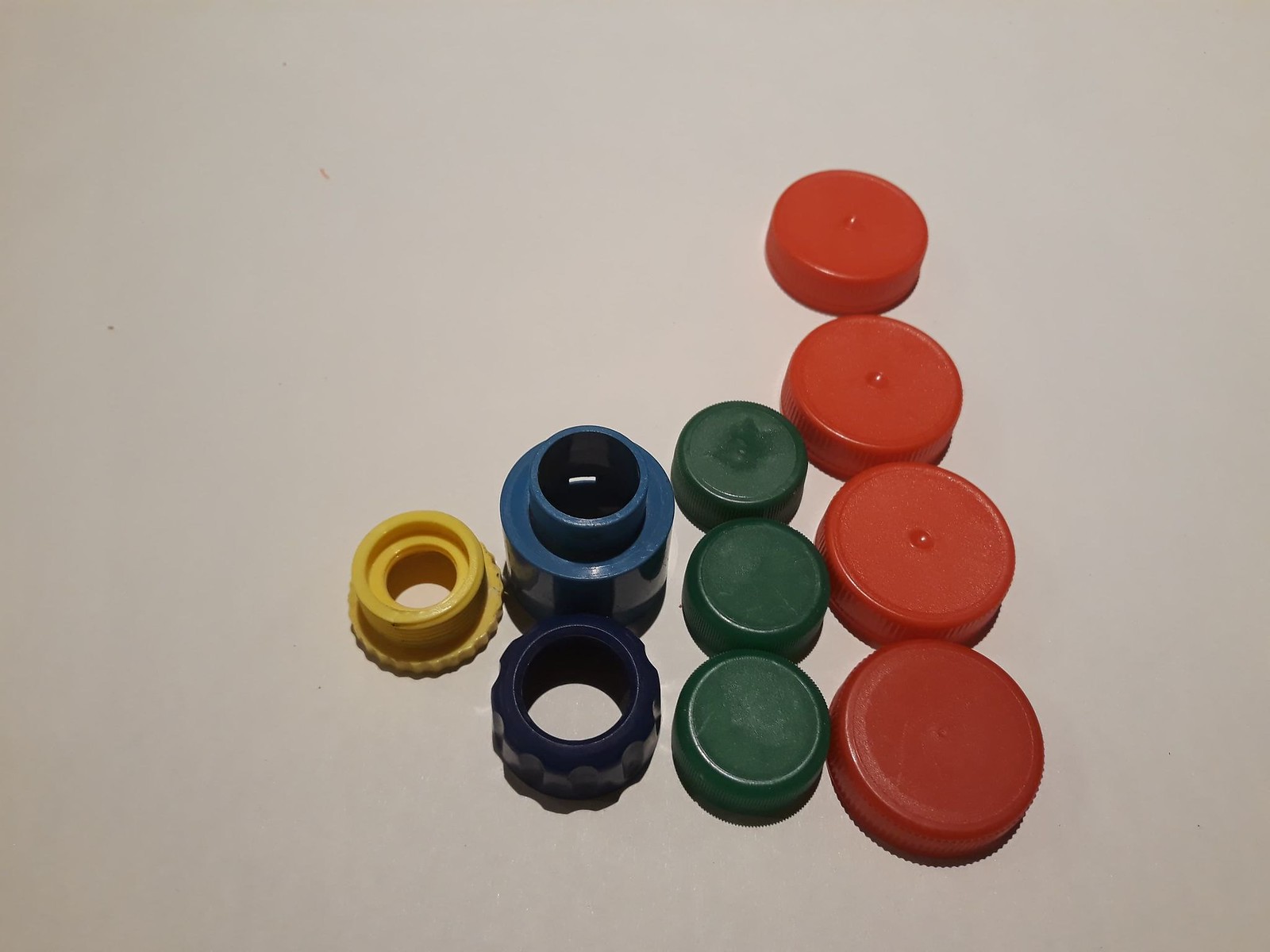The image showcases an array of various colored caps and components, organized into four neat rows on a bluish-white background. To the far right, there are four large red caps with ridged edges, which resemble those of peanut butter jar lids. Next to them, three smaller dark green caps are aligned vertically. Adjacent to the green caps, there are two blue cylindrical components with ridges around the edges, appearing to fit together. To the left of these, a single yellow component with a washer-like design and a gear knob at the bottom is positioned, suggesting it might be part of a mechanical assembly. Additionally, there is a black cylinder with knobs around its exterior that looks like it can be screwed into place, possibly part of a valve assembly. The overall arrangement presents a variety of plastics parts, possibly lids and machine components.